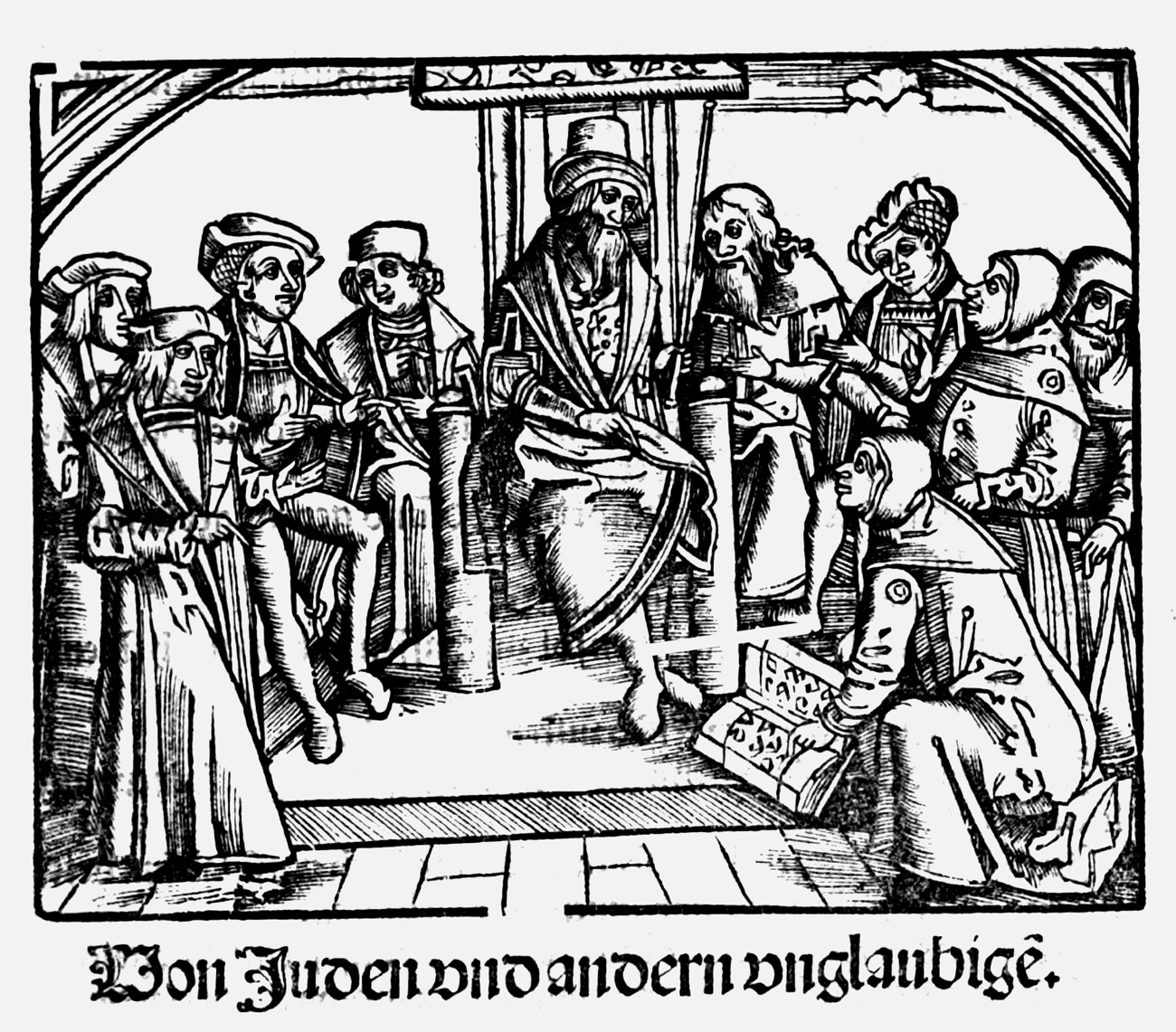The image is a detailed black and white medieval-style woodcut or drawing featuring ten figures dressed in period attire, reminiscent of military and monk clothing. The central figure, a bearded man in a long robe and top hat, sits authoritatively on a throne that rests on a pedestal. Surrounding him are nine other individuals, some in medieval armor and others in elaborate, layered medieval garments, including a woman with a traditional wimple. The composition suggests a scene of significant historical or religious importance, with most of the figures' attention focused on the man on the throne. On the bottom right, one person kneels, holding an open book with illegible writings, possibly offering it to the group. The text in the image, rendered in a German script called Fraktur, reads "Von Juden und anderen Ungläubigen," translating to "Of Jews and other unbelievers." The scene captures a moment perhaps of preaching or a declaration, adding to its historical narrative.